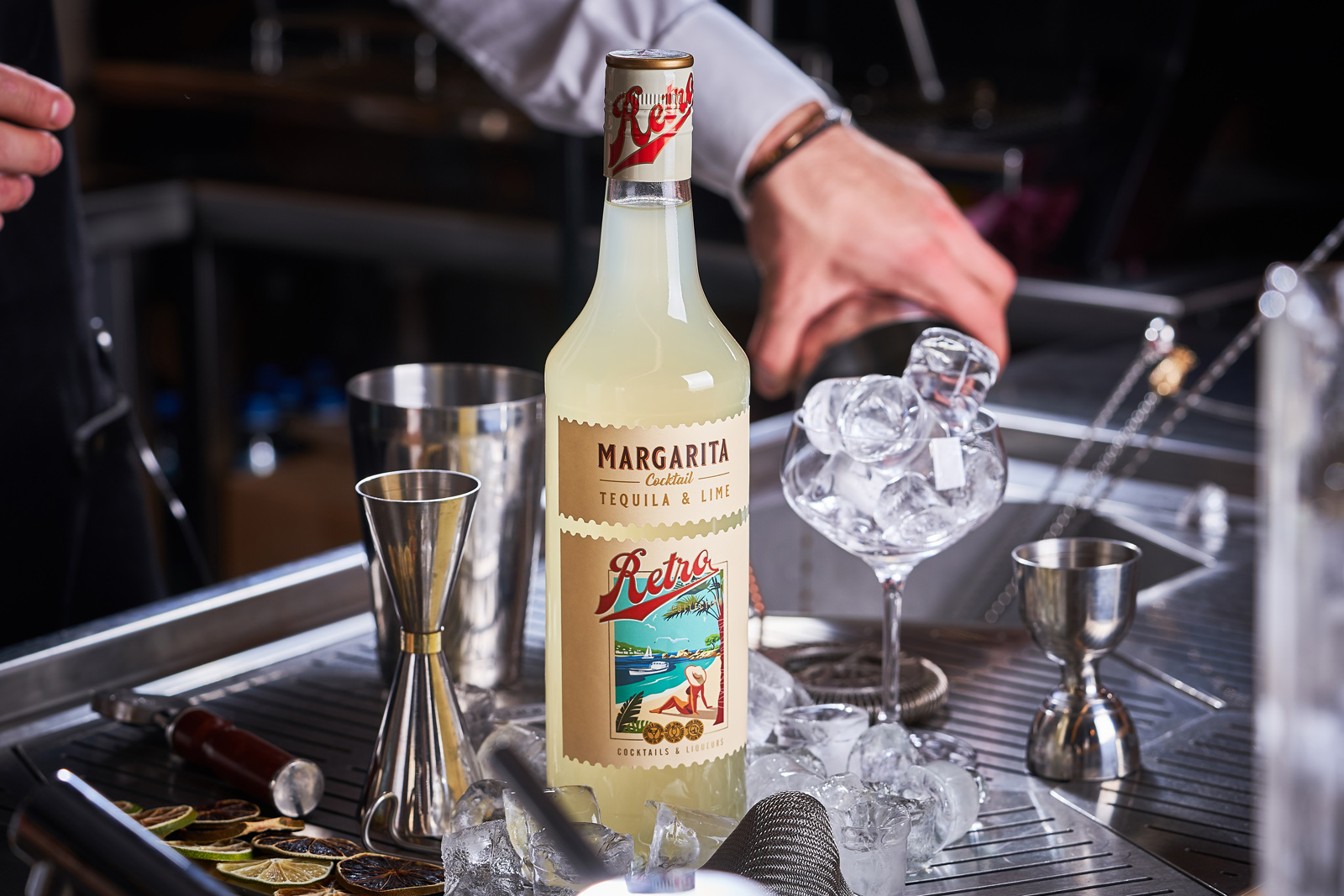In this detailed image of a beverage bar, a stainless steel counter takes center stage, showcasing a bustling scene of cocktail preparation. A sink is embedded within the counter, flanked by an array of bartending tools, including measuring cups and a knife. To the left, fresh lemon slices are neatly arranged, ready for use. A prominent hand, clad in a white shirt with the sleeve rolled up and adorned with a copper bracelet, grasps a mixing glass. This left hand suggests the presence of a bartender at work, while the right hand is partially visible in the upper left corner, poised and ready to assist. In the foreground, a martini glass brims with ice cubes, some of which have tumbled onto the counter. Adding to the scene's vivid detail is a clear bottle of margarita cocktail mix, positioned invitingly among the bartending ensemble, hinting at the delicious drinks being crafted.